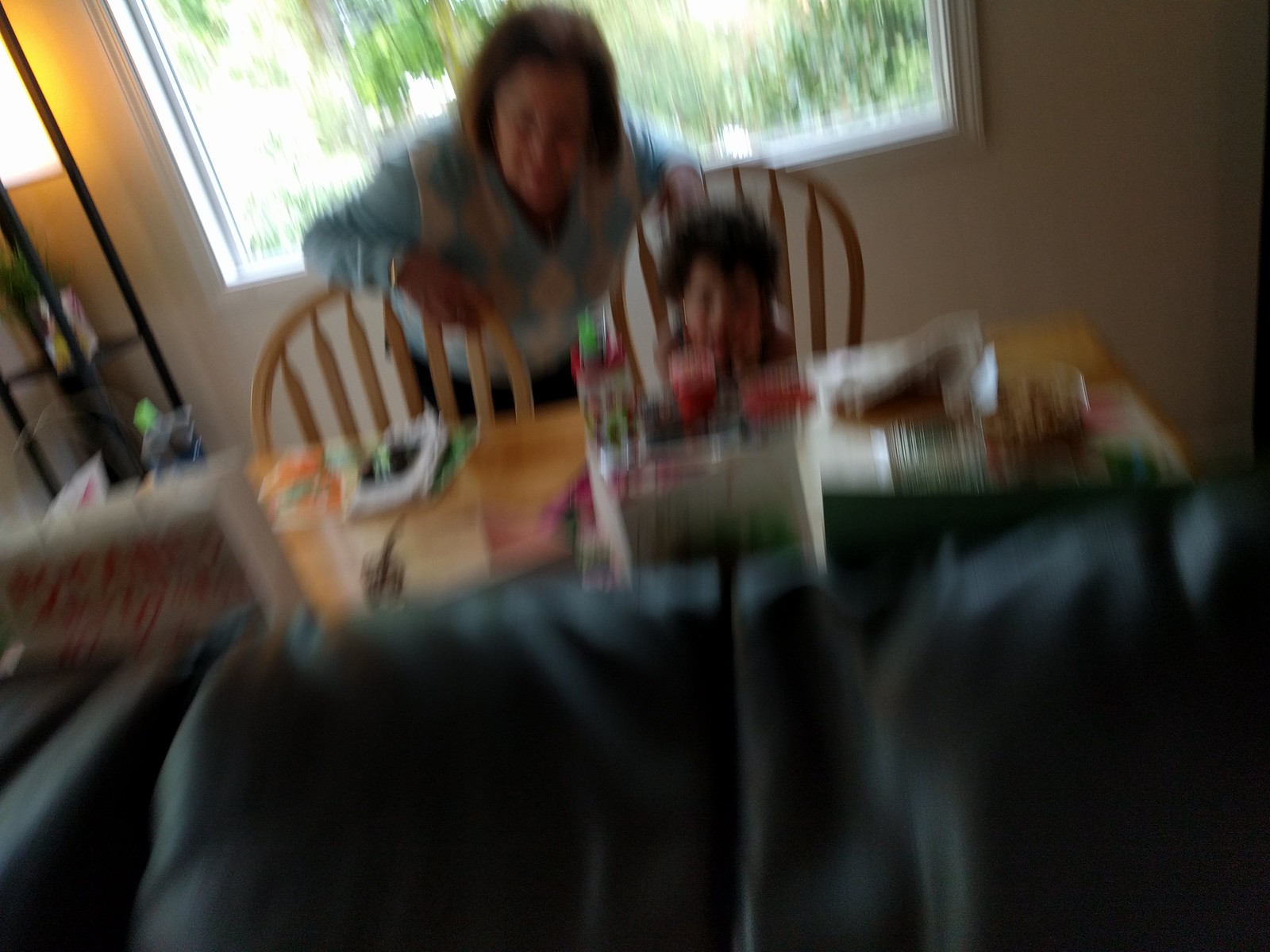In this very blurry photograph, we're given a glimpse into what appears to be a living room or dining room, showcasing a cozy and intimate moment. The primary focus is a large, wooden dining table set with two medium-colored wooden chairs featuring spindle backs and curved frames. Leaning over the chairs is a woman with fair skin and brown hair, dressed in a light blue long sleeve shirt and a sweater vest that has a blue and white diamond pattern. She is wearing a gold watch and appears to be engaged with the photographer. Sitting in the chair to the right is a young child with brown, curly hair, who also appears to be looking towards the camera. The table itself is cluttered with various unidentified objects, possibly cups, papers, or gifts, hinting at a dinner or craft event.

In the foreground, a black leather couch takes up about a third of the image, adding to the room's comfortable atmosphere. The room has off-white walls and features a large window without coverings, through which green foliage can be seen, bringing an element of nature inside. To the left side of the image, a square-shaped, black metal lamp with shelves adds a touch of modernity. Overall, despite the blur, the image captures a charming, everyday moment that exudes warmth and familial connection.